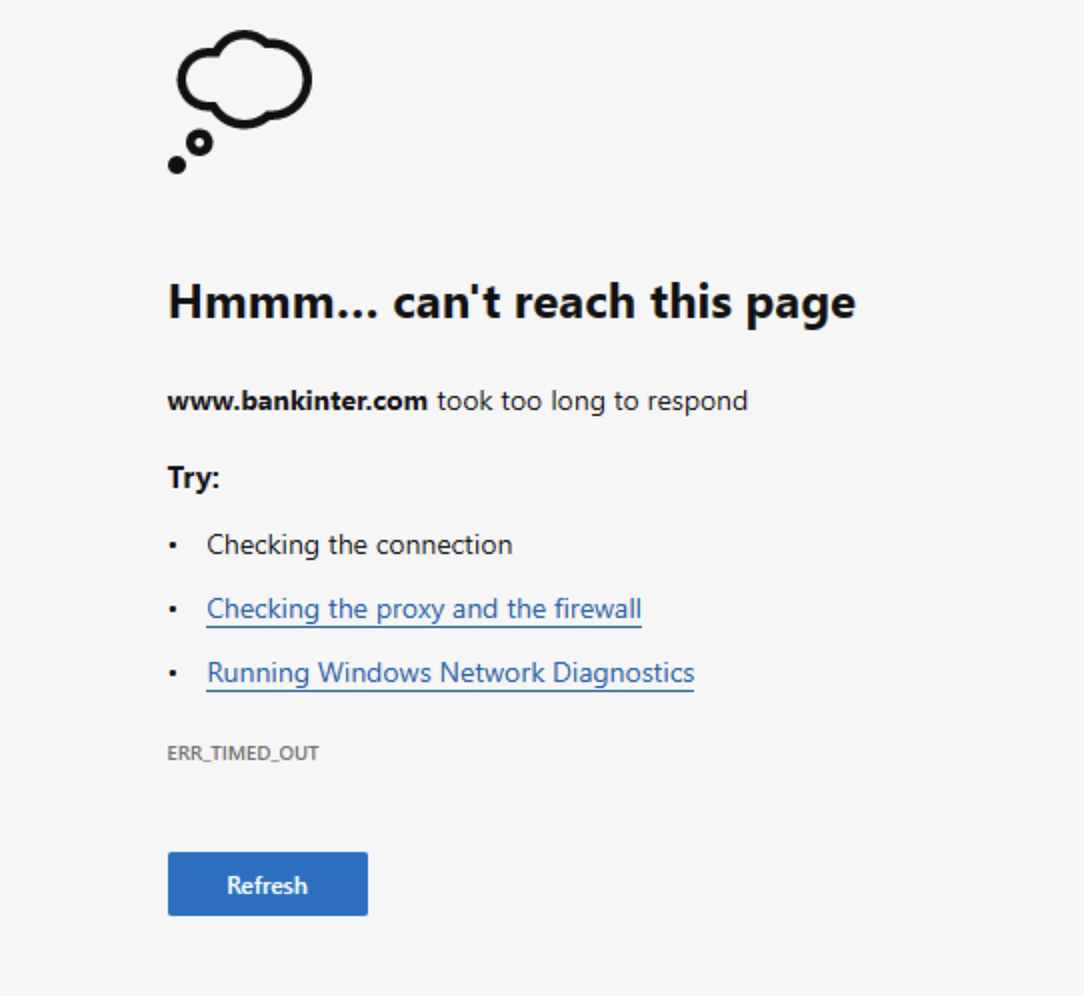The error page features a light gray background, entirely barren with no content on either the left or right sides. Centered on the page is an outlined black cloud. Below the cloud to the left is a black circle with a white center, alongside another solid black circle. 

About an inch below this illustration is the bolded text "HMMM..." in large black letters, followed by the phrase "can't reach this page" in smaller black font. Directly under this text is the URL "www.banktinker.com" in bold, accompanied by the message "took too long to respond" in regular font.

Further down, in bolded black text is the word "Try." Below this, aligned to the right of a black dot, is the instruction "checking the connection" in regular black font. A line lower, aligned with another black dot on the left, is the phrase "checking the proxy and firewall" in blue, underlined text. Next, on the following line, another black dot precedes the phrase "running Windows diagnostics," also in blue, underlined text. 

Finally, toward the bottom of the page, the error code "ERR_TIMED_OUT" appears in all capitalized black letters. Positioned about an inch below this is a light blue tab with the bolded white text "Refresh."